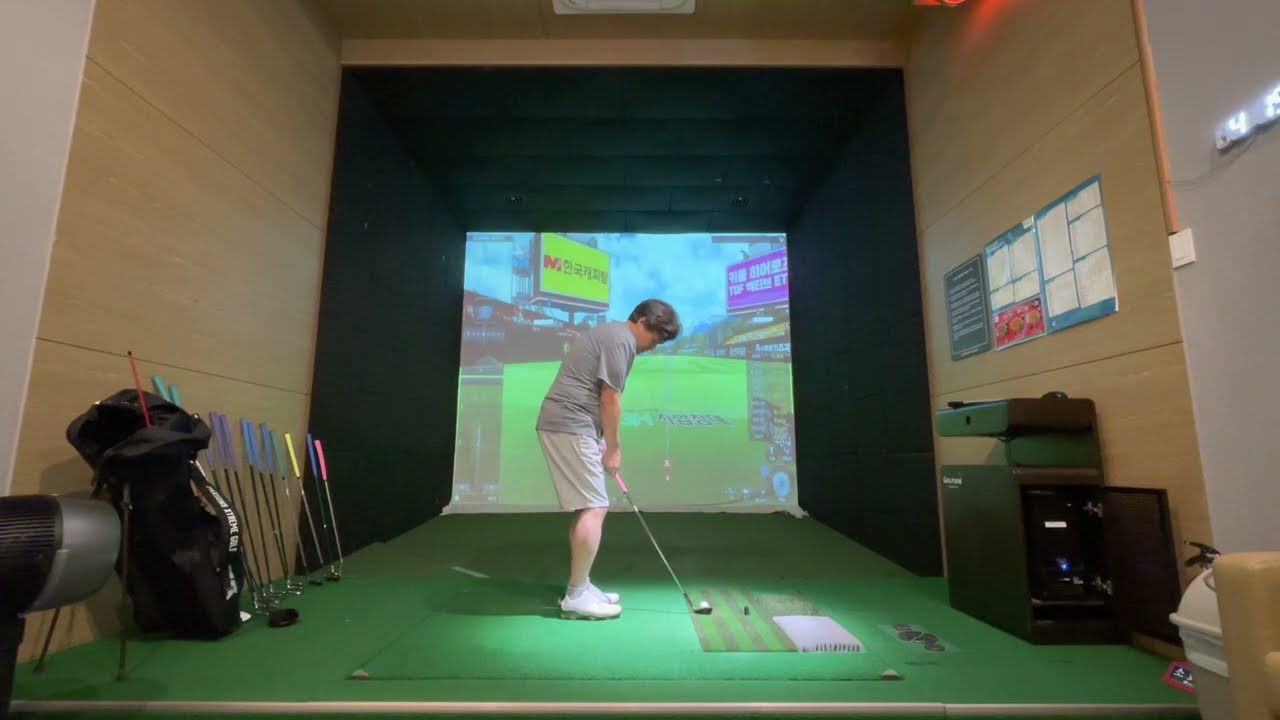A man, appearing to be Caucasian with short dark brown to gray hair, is standing on green artificial turf at an indoor putting course. Positioned sideways to the camera and crouched down, he prepares to tee off on a white golf ball at his feet. He wears a plain gray shirt, light gray shorts, and white shoes. His hands grip a golf club with a pink handle, and the club head is black. The floor, near the golf ball, features a pattern of green and black stripes.

In the background, a large animated screen displays a CGI golf course complete with green turf, a blue sky, and various billboards with yellow and purple backgrounds and white text. Light brown, wooden walls frame the left and right sides of the room. On the left side, several golf clubs with colorful handles (including pink, purple, blue, and yellow) lean against the wall, alongside a black golf bag. On the right side, three posters are pinned to the wall above a projection machine, which consists of a large black box with a green component on top. Additionally, a small cream-colored wastebasket can be seen at the bottom right of the image. The overall scene suggests an indoor setting designed for practicing golf swings, possibly located in a golf or sporting goods store.